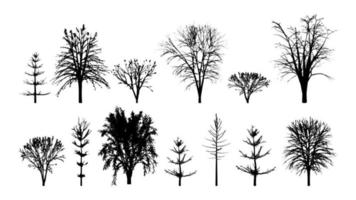The image, rendered in black and white, features meticulously detailed sketches of plants arranged in two horizontal rows against a plain white background. The top row showcases six different plants, while the bottom row displays seven. Each plant bears a unique structure, with some resembling spaced-out fir trees, others taking on the form of traditional oak trees, and a few appearing more like small bushes or bouquets. The depictions range from those with a singular stalk adorned with branches or leaves to sprigs of trees that might remind one of a Charlie Brown Christmas tree with additional limbs. Despite their tiny size making intricate details hard to discern, the variety in size, shape, and texture of these plant drawings is evident, bringing together a collection of botanical illustrations that blend the familiar with the abstract.